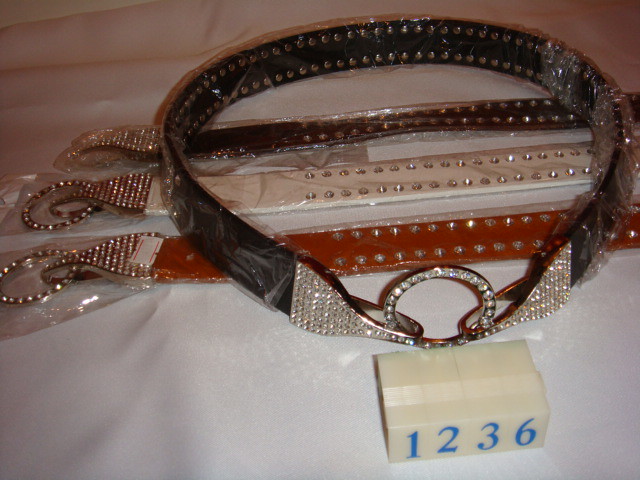The image showcases a collection of four belts arranged on a white background, possibly a sheet. Three of the belts are laid out flat, fully displaying their designs. The top belt is black, the middle one is white, and the bottom one is a brownish-orange shade. All three belts are adorned with two rows of sparkling rhinestones, including rhinestone-decorated belt loops. 

Another black belt is positioned above these three, clasped in a circular manner as if ready to be worn, with its rhinestone-studded buckle prominently visible. A piece of white paper lies beneath the belts, displaying the numbers "1, 2, 3, 6" in blue ink, suggesting a sequence or categorization. The paper appears to be slightly folded, adding to the overall composition of the image.